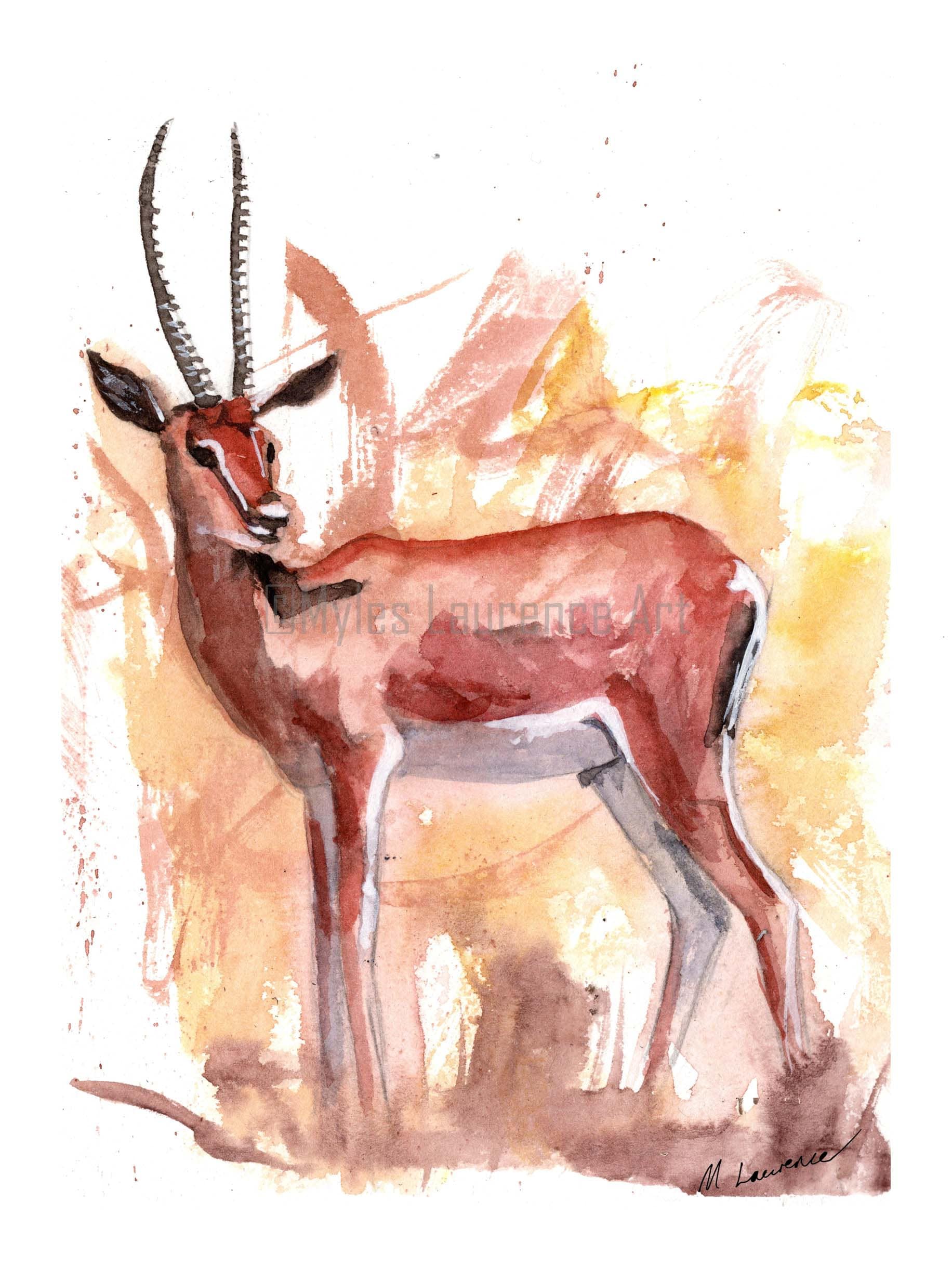This is a highly detailed watercolor painting by Miles Lawrence, depicting an antelope with distinct features. The antelope, a burnt orange-red, has a white underbelly and a white and black tail. Its body is angled to the left, but its head is turned to the right, showcasing its tall, striped horns and alert black ears. The antelope's lower legs blend seamlessly with the sketchy, brown soil, creating a cohesive transition. The background is an abstract mix of yellow, light brown, gold, pink, and hints of purple brushstrokes, giving it a warm, dynamic atmosphere. The painting is signed "M. Lawrence" in the bottom right corner, and also carries a watermark reading "Miles Lawrence Art." The subtle lighting suggests an unseen sun shining from above.